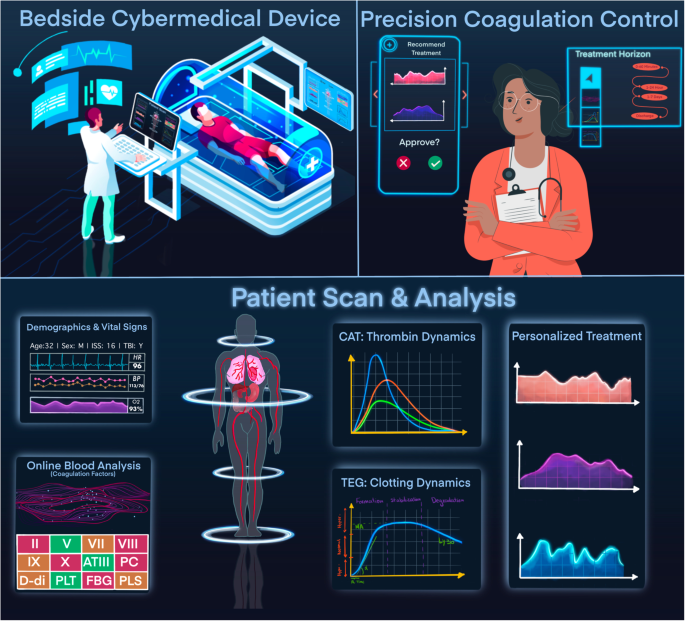The image is a detailed cartoon infographic divided into three distinct sections, each illustrating different healthcare procedures. The top left panel, labeled "Bedside Cyber Medical Device," depicts a male patient lying in a tube-like blue chamber, while a doctor stands beside a computer with multiple holographic screens displaying data. This doctor appears focused on monitoring the patient's condition. The top right panel, titled "Precision Coagulation Control," features a female doctor in an orange shirt with a stethoscope, examining various interfaces with options to approve treatments, indicated by checkmarks and crosses. She is surrounded by screens displaying charts labeled as Recommend Treatment Approve and Treatment Horizon. The bottom panel, which is the largest, is labeled "Patient Scan and Analysis." This section shows an x-ray view of the patient's circulatory system, surrounded by colorful charts that provide detailed metrics such as thrombin dynamics, clotting dynamics, CAT, online blood analysis, demographics, vital signs, TEG, and personalized treatments, giving a comprehensive look at the patient's health data.